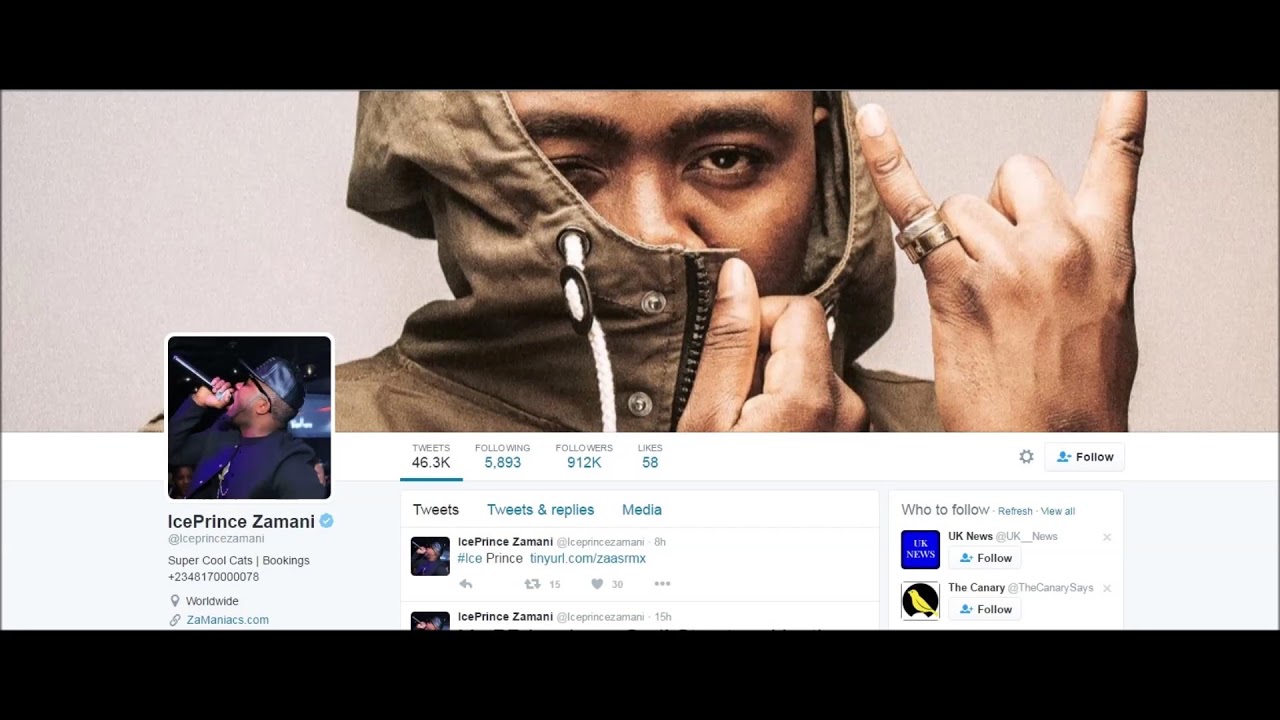This is a detailed screenshot of Ice Prince Zamani's Twitter profile. The top portion of the image features a close-up of Ice Prince Zamani, a well-known rapper. He is dressed in a brown coat with the hood pulled up, covering most of his face except for his left eye, part of his nose, and part of his eyebrows. His pose is highlighted by a hand gesture resembling the devil horns, with his pinky and index fingers extended and donned with rings. The image provides a glimpse into his social media activity, including tweets, followers, and following count. Additionally, there are design elements typical of a Twitter profile, such as a black border framing the page. The profile details prominently display his name "Ice Prince Zamani" along with his tagline "Super Cool Cats Bookings Worldwide" and the website "Zamaniacs.com." The color palette of the profile image includes shades of brown, olive green, white, blue, yellow, black, and gray. The snapshot effectively captures the essence of his persona and online presence.